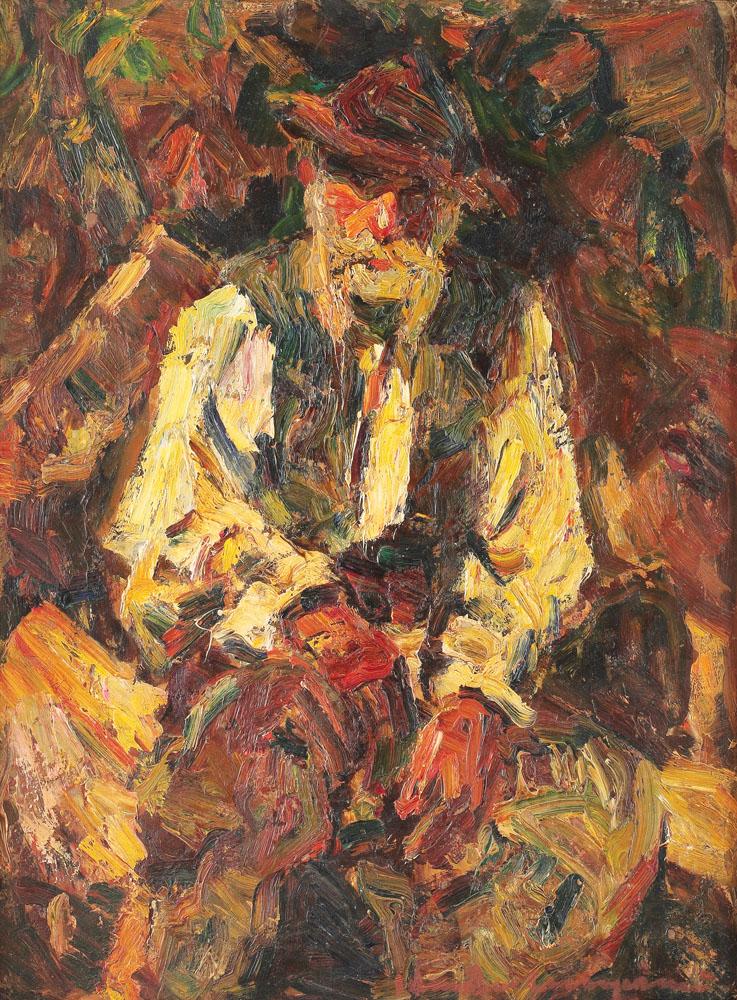This impressionistic oil painting, titled "Mose Gheorghe" by Rudolf Schweitzer Campana from 1940, portrays an elderly man seated against a backdrop of blended browns, greens, blues, and reds. The man, with his rosy cheeks and a red nose, sports a white beard and wears a low-profile, wide-brimmed brown hat. His attire includes a long-sleeved light-colored shirt under a blue vest and brown pants. He sits with an expressionless face, his hands resting on his legs, giving a tired, distant gaze. Though the painting's abstract style with blurred, opaque brushstrokes makes it hard to distinguish fine details, the man's eyes stand as the focal point, reflecting the power of this impressionistic portrait amid the muted, colorful background.